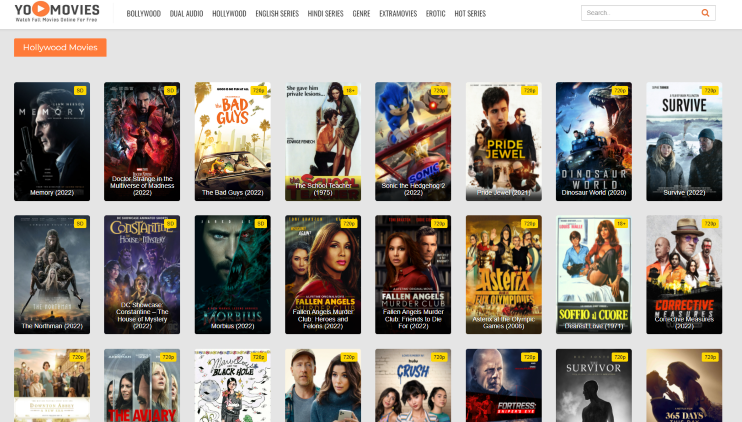The image displays an interface titled "Yo Movies," prominently featuring an orange circle with a white arrow pointing to the right in the center of the title. Below the title, partially legible text reads, "Watch Something Movies for Free." Despite the low resolution, the message suggests free movie viewing. 

On the right side, various tabs categorize content by genres and types, including Bollywood, Dual Audio, Hollywood, English Series, Hindi Series, Genre, Extra Movies, Erotic, and Hot Series. A search bar with an orange magnifying glass icon is visible for user queries.

The section below, labeled "Hollywood Movies," features an orange button. The interface showcases three rows of movie posters, each row containing eight posters. Some of the highlighted movies include "Memory," "Doctor Strange," "The Bad Guys," "Sonic 2," "The School Teacher," "Pride Jewel," "Morbius," "Constantine," "Corrective Measures," "Survive," and "Dinosaur World."